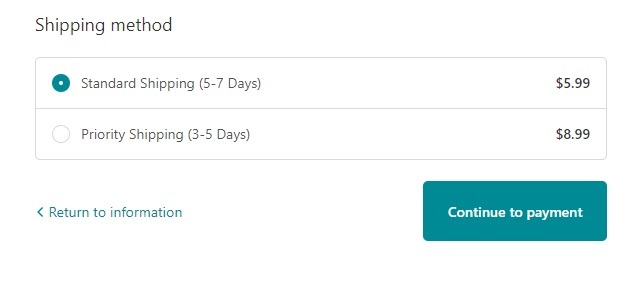This screenshot captures a user interface for selecting a shipping method, set against a solid white background. In the upper left corner, gray text labels the section as "Shipping Method." Below this, within a light gray outline, there are two available options arranged in two lines.

The first line features a teal-colored circular button, indicating that this option is selectable. To the right of the button, the text reads "Standard Shipping, 5 to 7 days, $5.99." Directly beneath, the second option is displayed: "Priority Shipping (3 to 5 days)," with the cost listed as "$8.99." This entire selection area is enclosed within a light gray border.

Below the shipping method section, on the left side, green text reads "Return to Information," accompanied by an arrow pointing left, suggesting a navigational option to go back to the previous step. On the right side of the screen, there is an action button labeled "Continue to Payment," suggesting the next step in the process. The interface is clean and minimalistic, ensuring clear visibility and ease of use for the user.